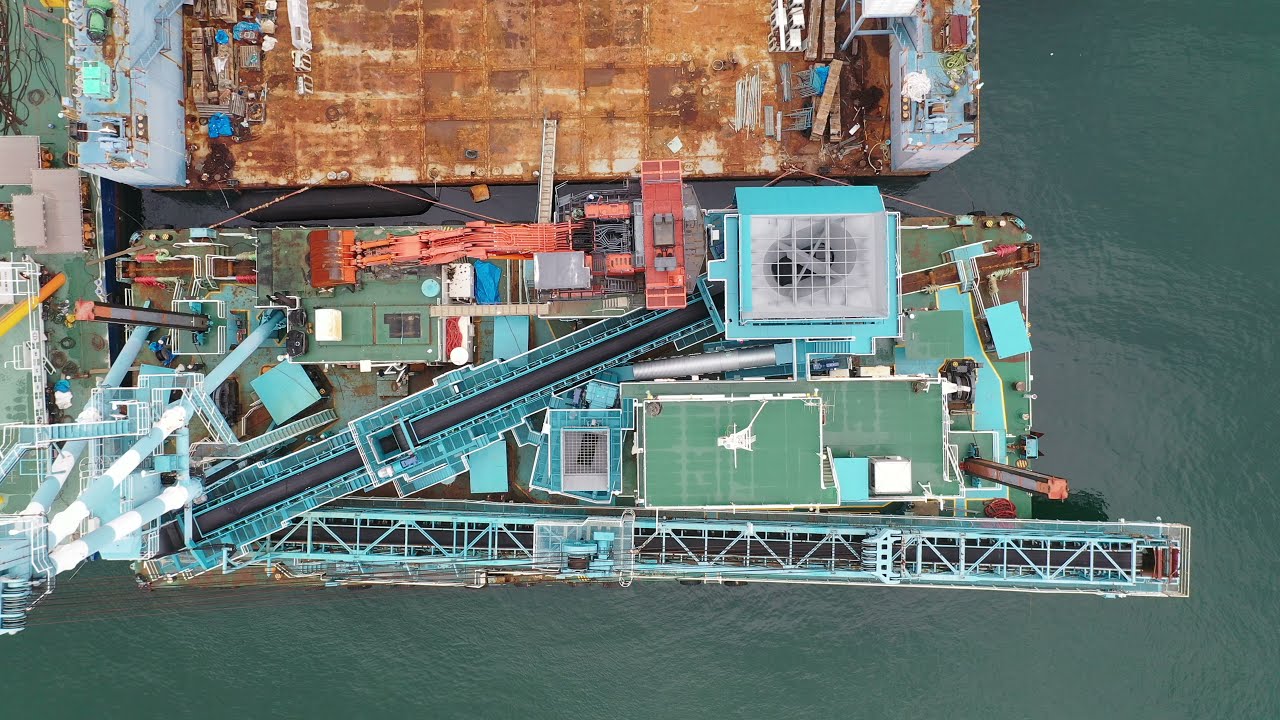The image is a detailed aerial photograph taken directly above a bustling industrial harbor. The focal point of the photograph is a large, rusty, brown barge with an empty cargo deck, positioned towards the top of the frame. Surrounding the barge, you can see the water, which has a dark greenish-brown hue, more prominent along the right side and the foreground. Just below the barge, there is an intricate network of mechanical structures, including cranes, tall metal objects, buildings, and trucks, all densely packed together. The cranes are colored blue and red, highlighting their industrial nature. Additionally, there is a second structure, possibly a pier or another vessel, situated in the bottom half of the image. This structure appears newer and cleaner, with a lot of visible machinery, pipes, and large tools. This complex scene vividly captures the bustling and industrious atmosphere of the harbor.